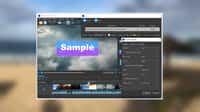A complex and visually intriguing image showcases a blurred beach scene with a distant ocean horizon under a blue sky. In the right-hand corner, a sunshade structure can be faintly discerned. Superimposed over this hazy coastal backdrop is another blurred image depicting a website interface. The website, primarily grey in color, features a left-hand pane that appears to be either playing a video or displaying a picture. Dominating the center of the website’s layout is a conspicuous button or label with the text "Sample" inscribed in white. This label stands out against a gradient background transitioning from blue on the upper half to purple on the lower half. Although the detailed elements of the image are vague, the overall impression is of a layered digital composition combining elements of nature and technology.